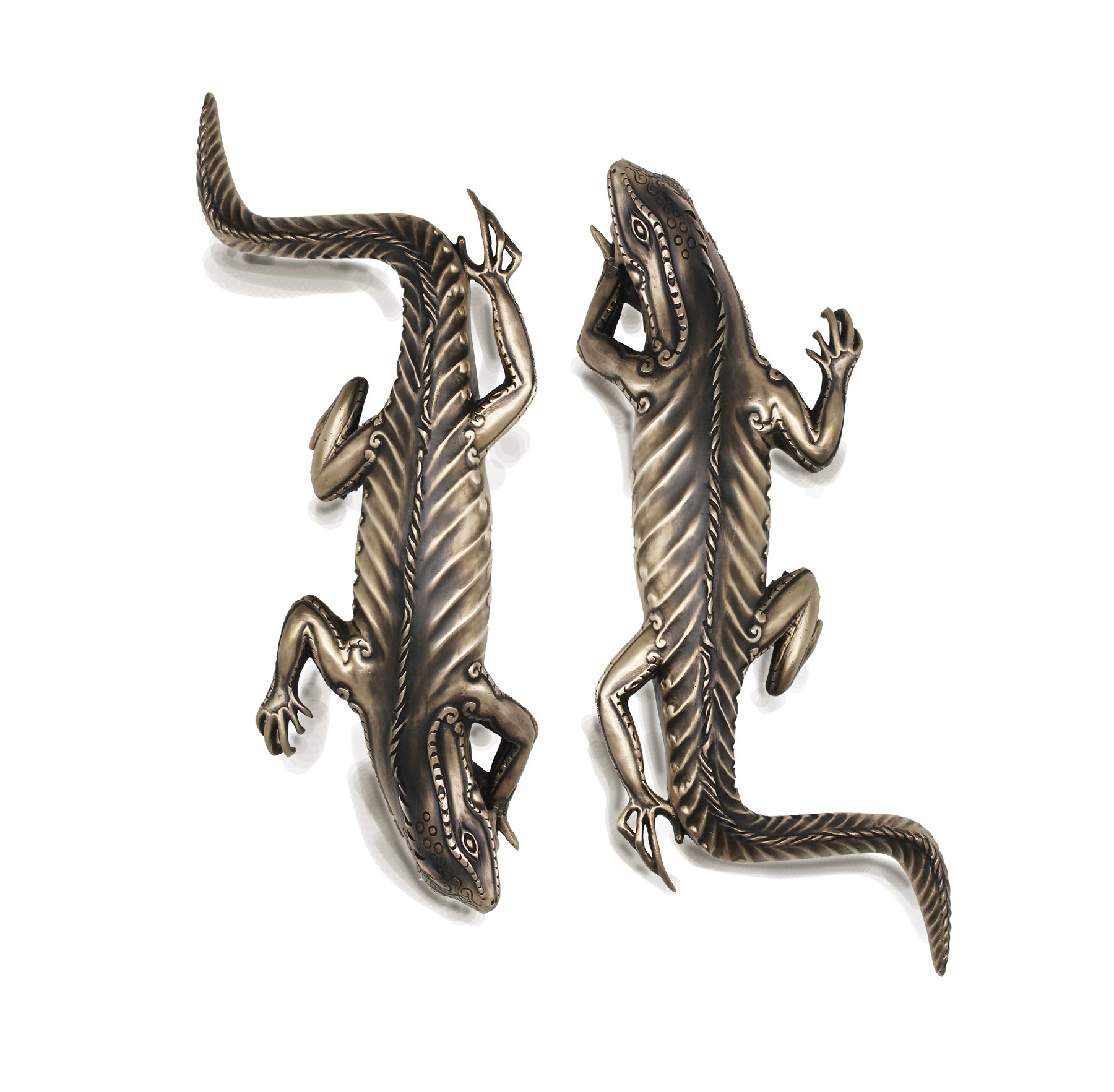This studio photograph features two intricately detailed metal salamander sculptures, posed against a plain white background. Both salamanders showcase a high level of craftsmanship, with etched, bumpy skin and extending claws, crafted from a material that could be silver, pewter, brushed bronze, or brushed nickel. Each salamander has a long tail and a pointy nose with visibly defined eyes. The left salamander faces downwards, while the right one faces upwards. They appear to be of identical shape and design, with each having one leg and arm extended forward and the others pulled back, creating a dynamic, lifelike posture. The exact scale of these pieces is unclear, though they are estimated to be around 14 inches long and may serve as decorative items for a home or garden. The dark brown coloration along the middle of their bodies adds to their elegant, metallic appearance.